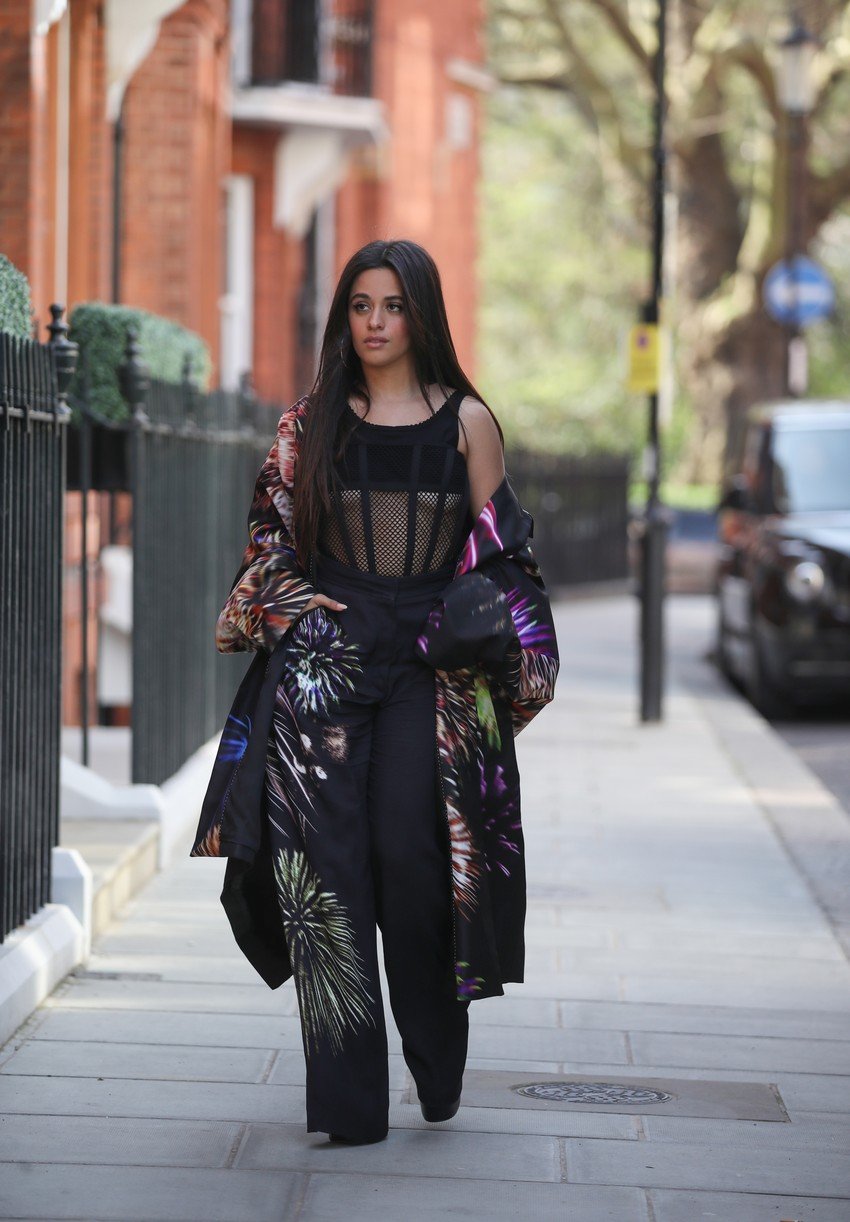The photograph captures a young woman with long dark hair and dark eyebrows walking toward the camera on a city sidewalk composed of gray stone slabs. She is passing a manhole cover to her left and a black rail fence that runs from the middle left of the image behind her to the right. The background features an orange brick building with iron fencing in front of it on the right, and a car parked near the curb on the left.

The woman is dressed in a striking black outfit detailed with a colorful firework pattern on her right pant leg in green and purple. Her black mesh top reveals the lower part of her breasts, and she dons an extremely colorful black cape, adorned with a similar fireworks motif, that falls off her shoulders and trails behind her. She appears to be holding the cape just around her arms. A metal pole is visible to the far right, extending out of the top of the image.